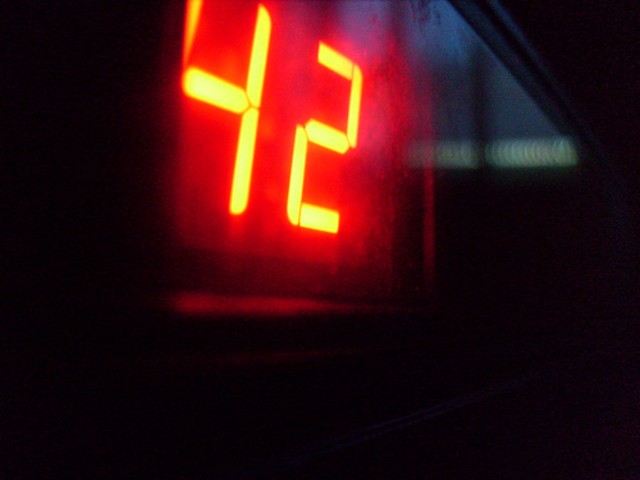This image captures a brightly illuminated digital sign displaying the number 42. The numbers, formed by straight lines like those on a digital clock or calculator, emit a vivid neon yellow glow. Surrounding the yellow digits is an intense, deep red light that stands out starkly against the predominantly dark, almost black background. The entire scene appears to be viewed through a window, suggested by a heavy diagonal black line in the top right—likely the window's edge. Reflections and distortions caused by the glass give the image a somewhat blurred appearance, particularly noticeable with the glowing numbers. In the left part of the image, faint reflections hint at three hanging blue fabric pieces with white borders, though these details remain indistinct. The background also features some round, coin-like shapes, further adding to the image's enigmatic composition.